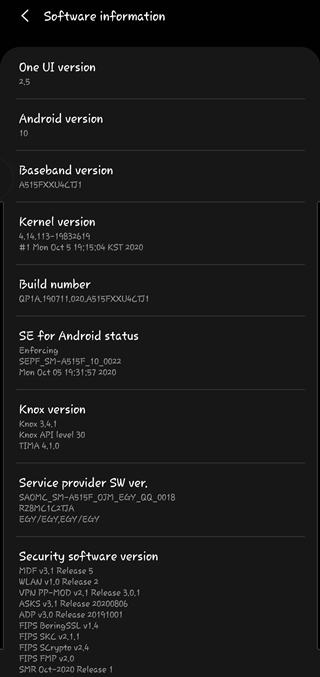A screenshot from a cell phone displaying detailed software information is featured in this image. The interface showcases an organized list of software-related categories presented in crisp, white text against a sleek black background. At the top, a less-than sign icon is visible, suggesting a navigation option to return to a previous screen. 

The detailed categories presented include "One UI Version" listed as 2.5, "Android Version" marked as 10, "Baseband Version" featuring a specific sequential digit number, "Kernel Version" noted as 4.14.113-14832614, "Build Number," "SE for Android Status," "Knox Version," "Service Provider SW Ver.," and "Security Software Version." Below each category heading, the corresponding version or status is displayed in white text. The image conveys detailed technical information about the device's software configuration, providing a comprehensive view of the system's specifications.